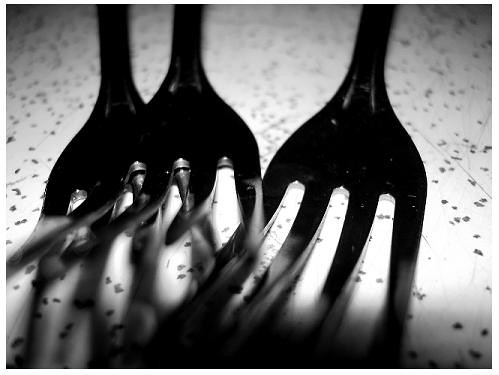This black and white photograph is a close-up shot of three four-pronged silver forks, each bent to varying degrees, creating an intriguing visual arrangement where they slightly touch each other. The middle fork is the most prominently bent. They rest on a surface that appears white and is scattered with black specks, resembling either confetti or paper scraps. The photograph focuses on the business ends of the forks, extending about half an inch beyond the prongs. The forks are partially in shadow, with light streaming in from behind but not fully illuminating them. This emphasis on shadow and light adds depth and contrast to the image, with the background remaining slightly blurry while the foreground forks are sharply defined.